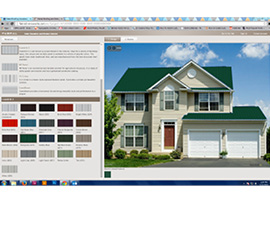The image depicts a two-story house displayed on a website that features a design function. The webpage is open in a windowed browser with multiple tabs, which are too small to read, situated at the top. The browser window is characterized by a collection of colorful triangles in shades of orange, light blue, dark blue, and white at the top and Windows icons in the bottom-left corner on a darker blue background.

The house itself boasts a green roof and a dual car garage divided by a slight split. The white garage doors complement the brown front door, which is fitted with a white storm door. On the left side of the exterior, the house exhibits a window on both the first and second floors. Additionally, there is a window above the front door and two windows above the garage. A paved driveway leads to the house, flanked by some shrubs and a partially off-screen tree. The background features a blue sky dotted with clouds.

On the left side of the webpage, several color options are visible, including reds, darker reds, light browns, greens, and grays, which are likely intended for customizing design elements such as the roof color or other aspects of the house.